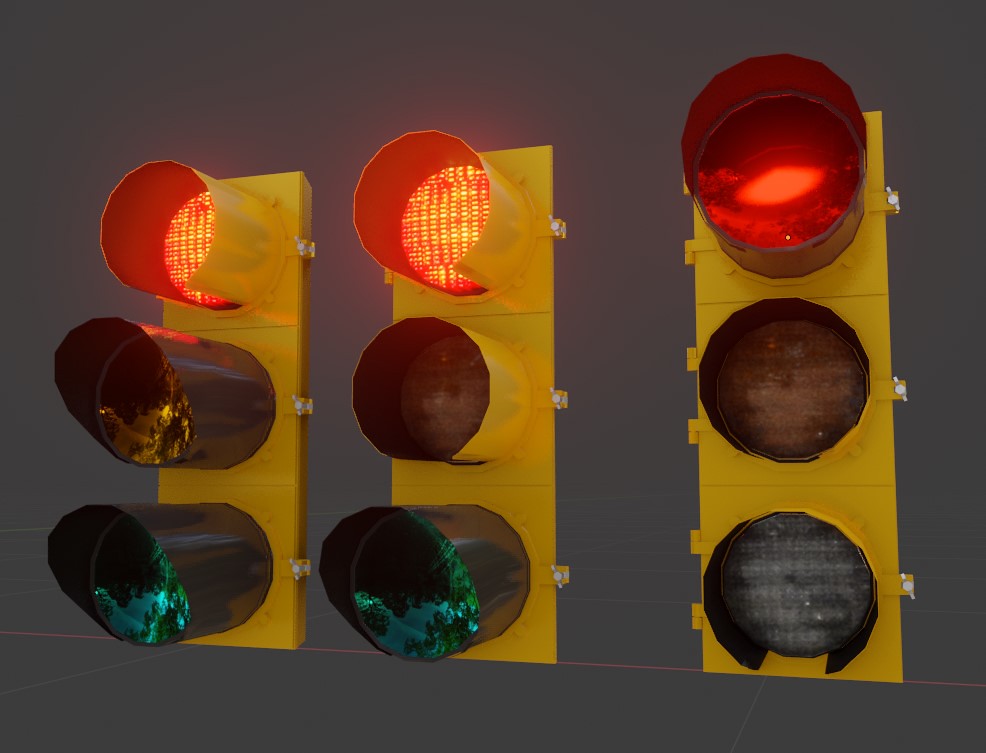The image depicts a digital rendering of three traffic lights, evenly spaced and aligned horizontally with a slight tilt to the left. The background is a solid gray, enhancing the vivid colors of the traffic lights. Each light has a yellow metal casing. The leftmost and center lights both have their red lights illuminated, with the center light featuring two yellow cylinders around the middle light and a blue cylinder around the bottom light. The rightmost traffic light also has its red light illuminated, but it appears dimmer than the others. The yellow and green lights in the left and center lights are not lit, while the rightmost light clearly shows no illumination for the yellow and green lights. The distinctive feature of this image is the uniform yellow housings and the specific colored cylinders wrapped around the lights.